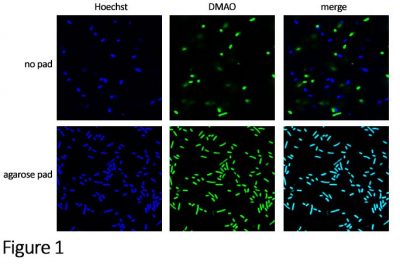The image shows a detailed scientific diagram composed of six sub-images arranged in a 2x3 collage format, each displaying a black background with fluorescent dots. The top row has three images, labeled from left to right as "H-O-E-C-H-S-T," "D-M-A-O," and "MERGE." The left-most column is labeled "No Pad" on the top row and "Agarose Pad" on the bottom row. The entire diagram is annotated as "Figure 1."

The top-left sub-image ("H-O-E-C-H-S-T") features a sparse distribution of small, blue fluorescent dots. In contrast, the bottom-left sub-image shows a denser collection of elongated blue fluorescent shapes, more worm-like compared to the top image.

The top-middle sub-image ("D-M-A-O") presents fewer, faint green fluorescent dots. Conversely, the bottom-middle sub-image displays a much denser array of elongated green fluorescent shapes, resembling worms or pills, indicating a significant increase in quantity and brightness.

The top-right sub-image ("MERGE") combines both blue and green fluorescence but shows relatively sparse distribution. The bottom-right sub-image reveals an abundant mix of blue and green elongated fluorescent shapes, much more pronounced and densely packed than in the top row.

Overall, the diagram appears to illustrate the differences in fluorescence between samples on a "No Pad" and an "Agarose Pad," under various staining conditions, highlighting the visual differences in concentration and morphology of the fluorescent entities.